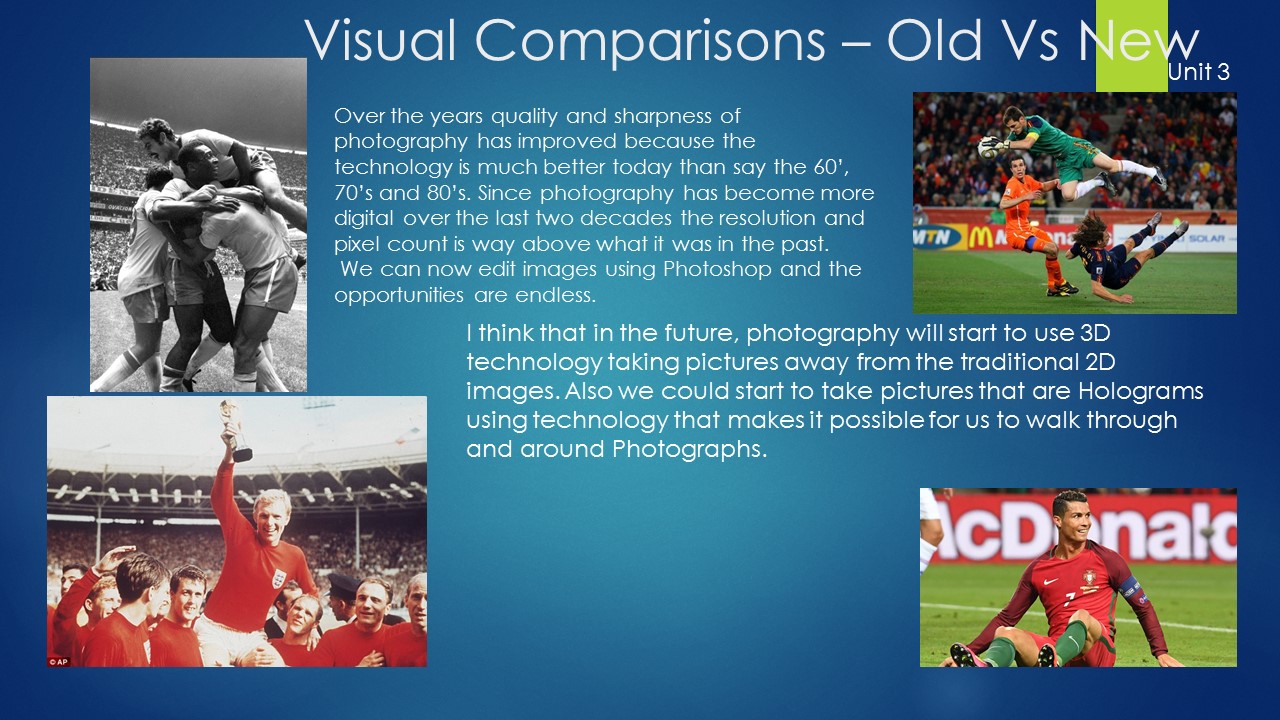This wide rectangular image is a detailed PowerPoint slide with a background that transitions from a light grayish-blue in the center to a deeper blue on the edges. At the top, slightly off-center, the main title in white font reads "Visual Comparisons - Old vs. New," followed by "Unit Three" underneath the word "New." In the top right corner, there's a green rectangle.

The slide features four photographs comparing old and new soccer scenes. On the left side, the upper-left photograph is a nostalgic black-and-white image of three soccer players huddled together with another player leaping above them. Beneath it, the second photograph shows a vibrant color image of soccer players wearing red shirts with insignia and white shorts. A young blonde player is being hoisted up by teammates, holding a trophy in celebration.

On the right side, the upper photograph captures a dynamic modern soccer scene with a goalie in a green uniform caught mid-air reaching for a ball, while another player in red attempts a move and a third, dressed in black, is falling to the ground. The background displays stadium stands with visible McDonald's advertising banners. The lower-right photograph depicts another modern scene of a player in a red uniform with green socks sitting on the ground, smiling in a profile view, as remnants of the McDonald's signage are partially visible behind him.

Between these sets of photographs are two paragraphs in white font. The first paragraph discusses the technological advancements in photography, stating how digital advancements have significantly improved image quality and editing capabilities. The second paragraph, in larger lettering, speculates about the future of photography, envisioning a shift towards 3D and holographic imaging. 

Overall, the image serves as an illustrative comparison of soccer through different eras, highlighting the evolution in photographic technology and its prospects.